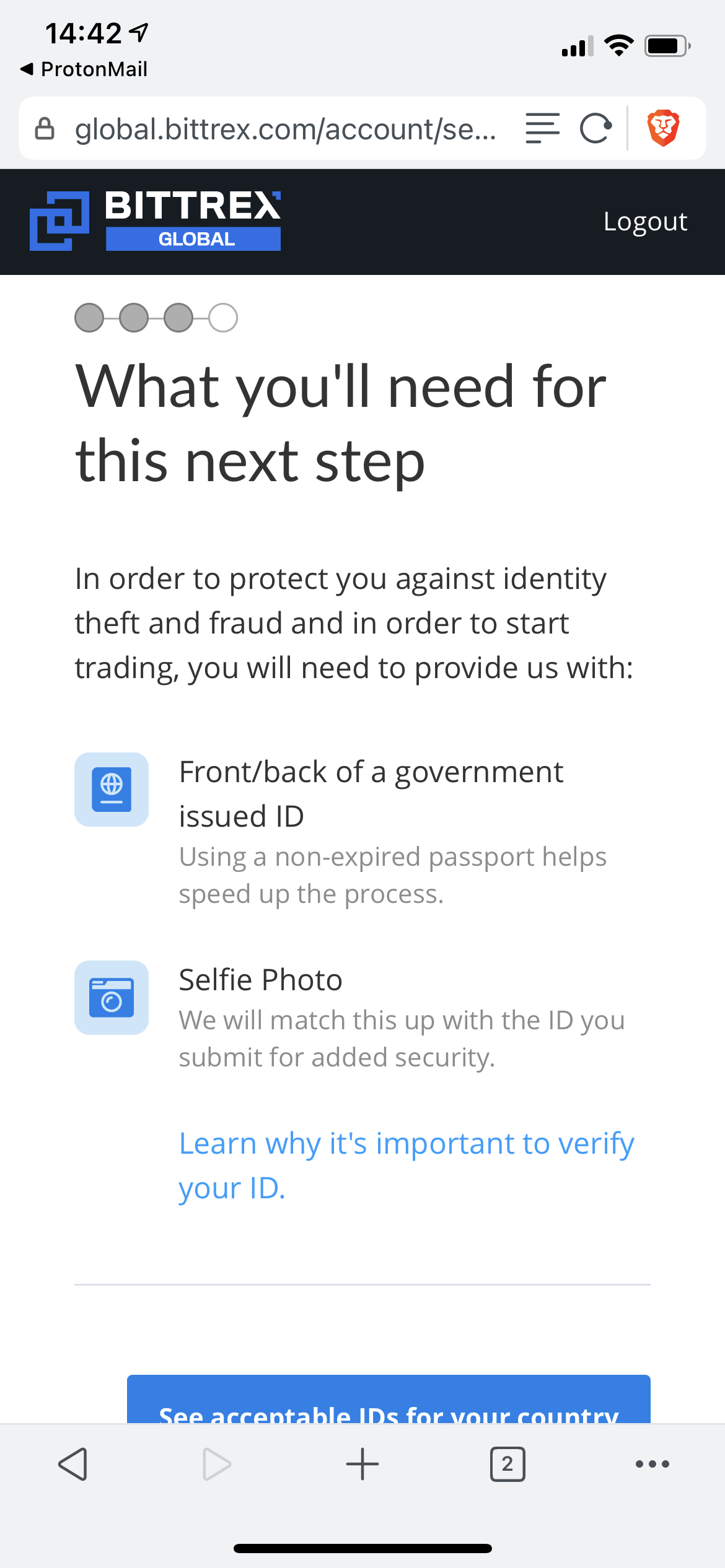This image is a screenshot from a mobile phone, showcasing a web page viewed through the Brave web browser, identifiable by its red lion logo. At the very top, there's a status bar displaying the time "14:42", next to a paper airplane icon, implying a notification from ProtonMail. Adjacent to this icon, the cellular signal strength is shown as three out of four bars, alongside a black battery symbol.

The web browser's address bar below it indicates the URL "global.bittrex.com/account/se...", hinting at a financial or trading website. Positioned to the right of the address bar are navigation icons: four horizontal lines for menu access and a circular arrow for refreshing the page.

Underneath, there's a black bar featuring an icon of two interlocking squares, with text reading "Bittrex Global Logout". Following this, the screen displays a sequence of four circles, with the first three filled in gray and the last one white, possibly indicating a stepwise process.

The main content of the page is geared towards user verification, with a header stating, "What you'll need for this next step." It explains that to protect users against identity theft and fraud, and to enable trading, users must provide the "front and back of a government-issued ID", emphasizing that a non-expired passport can expedite the process. Also required is a "selfie photo" for added security by matching it with the submitted ID. Below this, blue text provides a link to "Learn why it's important to verify your ID."

At the very bottom, there is a partially obscured blue button, with the discernible text hinting it says, "See acceptable IDs for your country."